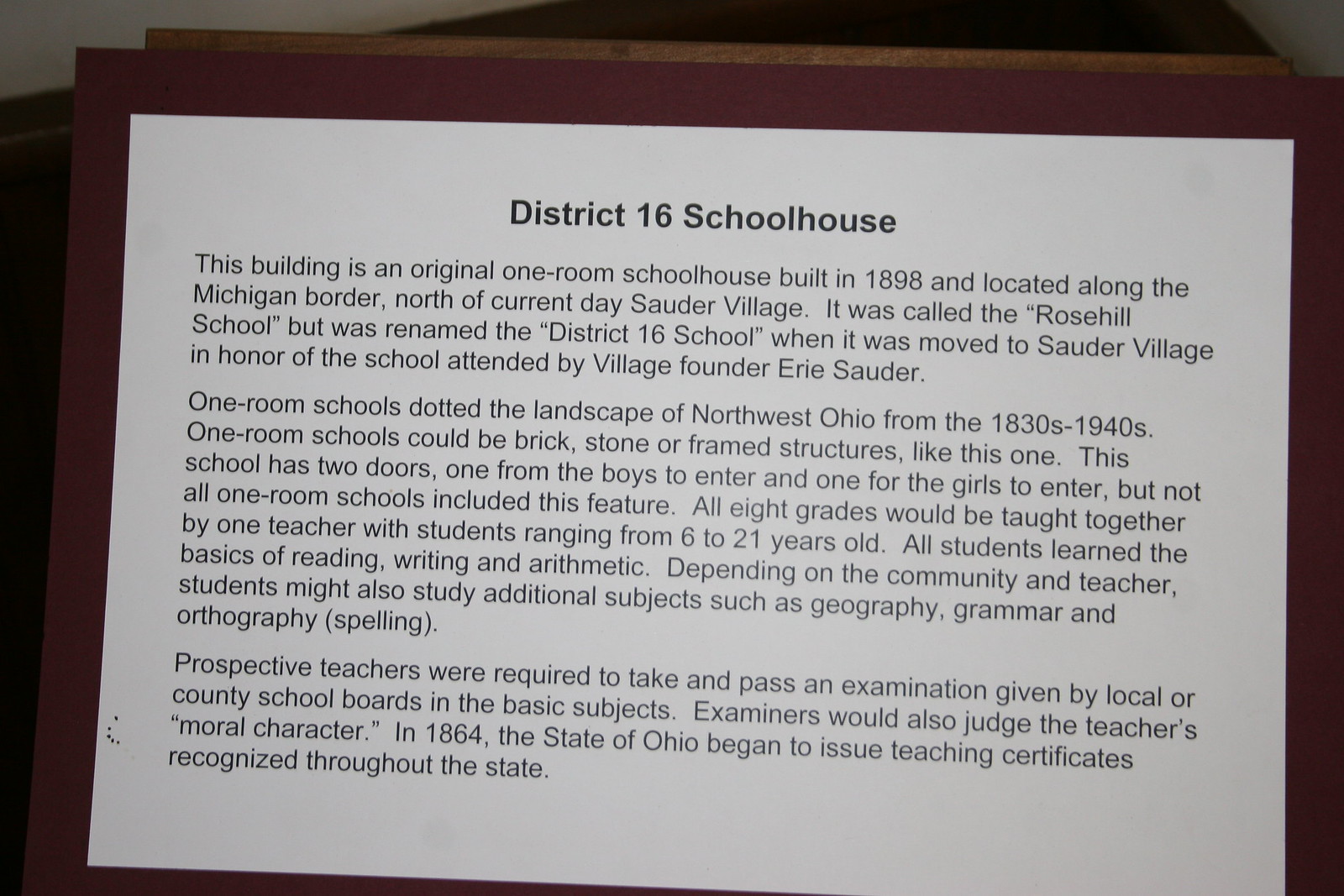The image features an informational sign or plaque, prominently titled "District 16 Schoolhouse" in bold black text at the top. The rectangle-shaped sign, primarily white, is bordered by a maroon background and is propped against a brown wooden platform. It includes three paragraphs of detailed black text. The first paragraph explains that the building is an original one-room schoolhouse, constructed in 1898 along the Michigan border, north of current-day Sauder Village. Initially named Rose Hill School, it was later renamed District 16 School upon its relocation to Sauder Village, in honor of the village's founder, Erie Sauder. The second paragraph describes the prevalence of one-room schools in northwest Ohio from the 1830s to the 1940s, noting that these structures could be built from brick, stone, or wood. This specific school features two separate entrance doors for boys and girls, a characteristic not found in all one-room schools. It also details that a single teacher taught all eight grades, with students ranging from 6 to 21 years old, covering basic subjects like reading, writing, and arithmetic, and potentially additional subjects depending on the community and teacher. The final paragraph outlines the requirements for prospective teachers in the area, including passing examinations given by local or county school boards in fundamental subjects and assessments of their moral character. It also mentions that Ohio began issuing statewide teaching certificates in 1864.